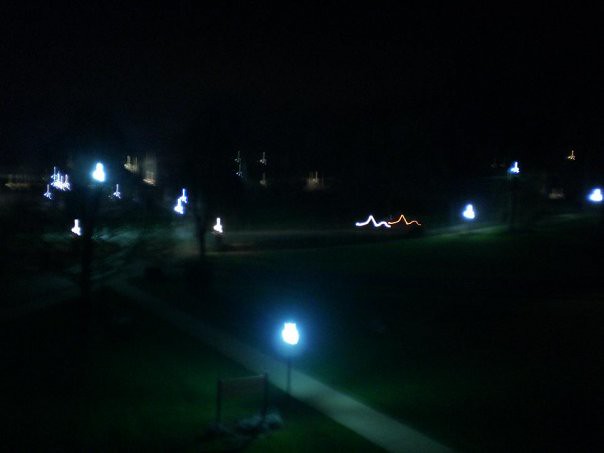A captivating scene unfolds in the darkness of night, showcasing a well-maintained park illuminated by numerous lights. The lush, green grass stretches across the hill, bordered by tidy sidewalks that crisscross the landscape. In the foreground, an old-fashioned lamppost casts a warm glow over a sign surrounded by carefully placed boulders, though the sign's text remains unreadable. In the distant corner, small, zig-zagging lights give an almost electric appearance, adding an enigmatic touch to the serene setting. The absence of people enhances the tranquility of this meticulously cared-for park, encapsulating the serene beauty of this nighttime scene.